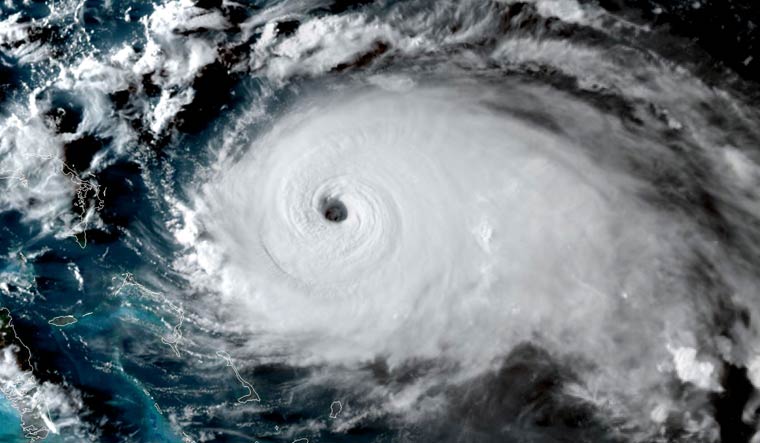This aerial satellite image, captured in vibrant color, showcases a direct overhead view of a formidable hurricane swirling over the ocean. The image is in landscape orientation, with the eye of the hurricane prominently positioned slightly left of center. The eye is depicted as a dark void surrounded by intense, thick white clouds. As these concentric clouds spiral outwards in a counterclockwise direction, they gradually thin and transition to a mix of lighter grays. The densest part of the spiraling cloud bands spreads predominantly to the right, tapering off near the edges of the image. Wispy peripheral clouds are visible particularly around the upper left and right corners. The scene vividly contrasts with the ocean below, where deep blue waters peek through the swirling storm. There are no evident landmasses, underscoring the hurricane's location over open water. This realistic satellite imagery provides a detailed and compelling view of the natural phenomenon from space.